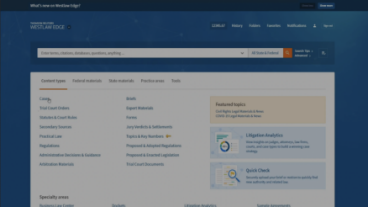This image captures a web page interface set against a visually degraded background, rendering the text largely illegible. The page features a prominently displayed search field, accompanied by several navigation links and dropdown menus. Distinct colors such as blue, orange, yellow, and white dominate the visual scheme, adding a vibrant yet somewhat obscured aesthetic. A cursor is visibly hovering over one of the interactive items, albeit the exact details remain indistinguishable due to the degradation.